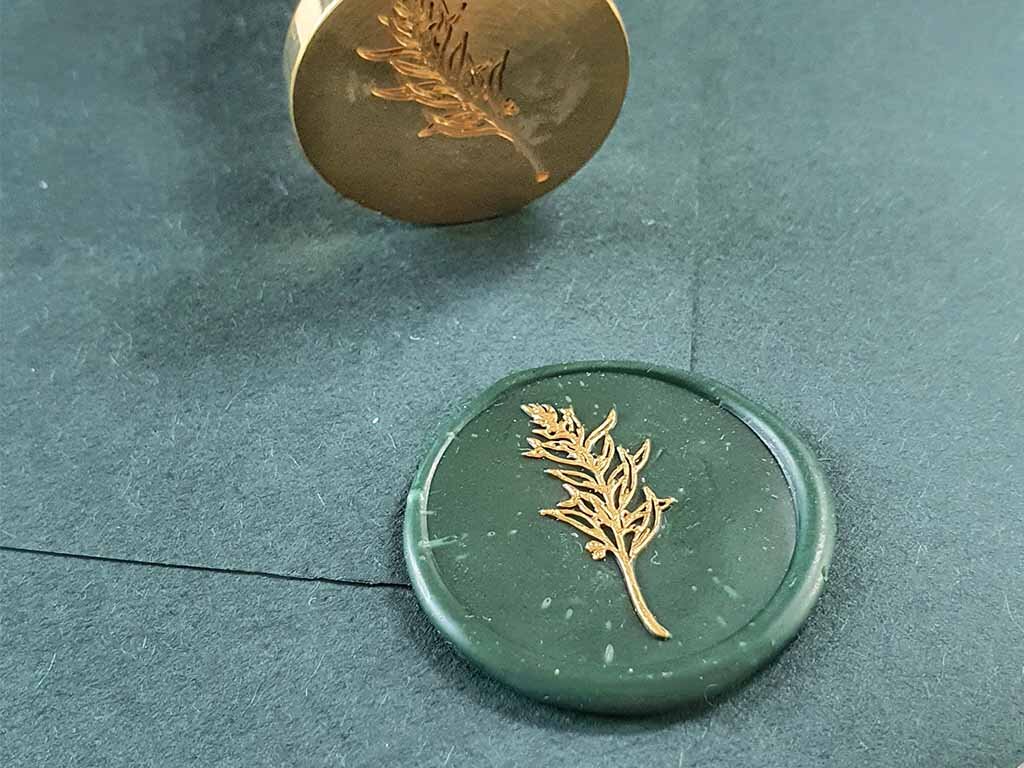A detailed, cleaned-up caption of the image:

"Displayed on a textured gray concrete surface, this art piece features a round green plate with a stylized 3D tree emerging from its surface. The tree, characterized by its long, wavy trunk and stylized leaves, is rendered in a striking gold color, creating a vivid contrast against the green background. The plate itself shows signs of discoloration, adding a touch of rustic charm. Hovering above the green plate is a gold-colored stamper, bearing an indented version of the same tree design. This stamper appears meticulously crafted, likely used to imprint the intricate tree onto the plate. The scene showcases a blend of modern 3D printing or molding techniques with artistic flair."